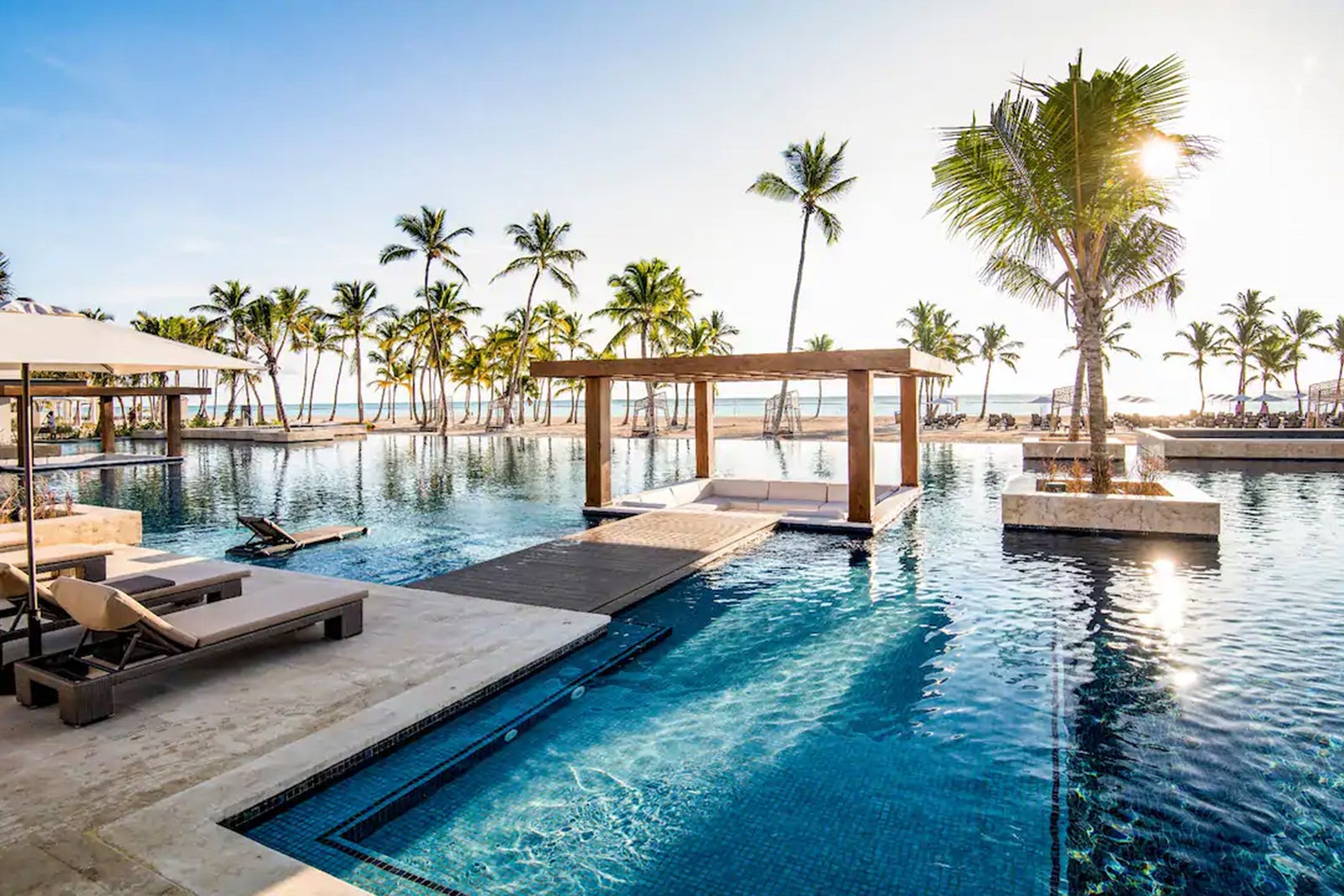A daytime photo of a serene, tropical beach resort featuring a vast, modern swimming pool with bright blue water. The pool includes a unique sunken seating area with soft, white couches surrounded by the water. At the right side of the image, two large palm trees appear to be floating in the pool, contributing to the exotic ambiance. The foreground showcases a well-appointed deck area with several chaise lounges and beige umbrellas, some of which are positioned directly in the water. 

Further back, a sandy beach stretches across the horizon, adorned with numerous palm trees that sit atop a sandbar, seamlessly blending into the deep blue ocean in the distant background. The bright blue sky and sun shining from the top right corner of the image illuminate the scene, enhancing the tranquil and inviting atmosphere of the resort. A charming gazebo or covered area with tables is visible on the left side, adding to the luxury and comfort of the setting. This picturesque image likely captures the beauty of a Caribbean island or a similar tropical destination, offering a perfect escape into paradise.